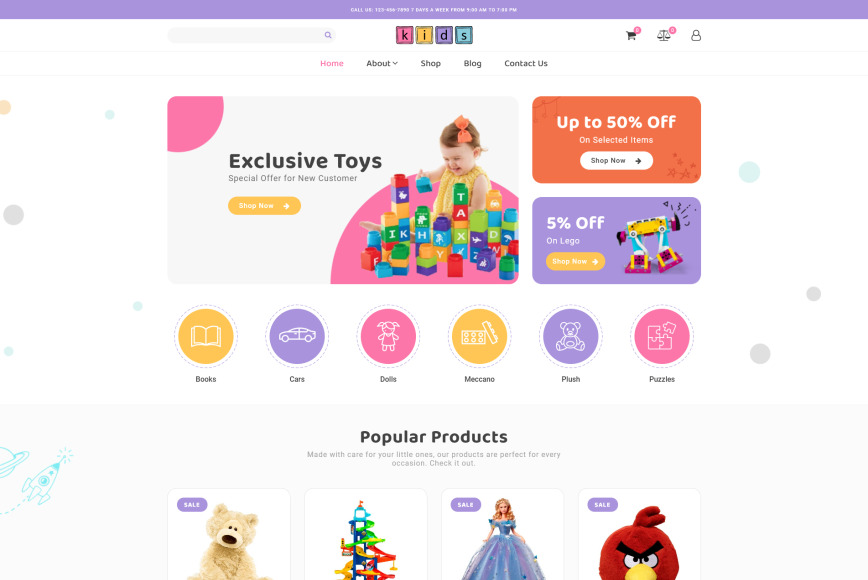**Detailed Screenshot Caption:**

The screenshot showcases a website layout, featuring a gray search bar at the top. Below the search bar, there are four colorful blocks, each in a different hue - pink, orange, purple, and teal. Each block contains a letter, collectively spelling out "KIDS." To the right of these blocks, there's a shopping cart icon with a red notification circle; although the exact number inside the circle is not legible. 

Further down, a balance scale icon with measurements marked on each side is visible. Additionally, another red notification circle with white numbers, also too small to decipher, appears nearby. A profile icon is present, likely for user account access. 

The main navigation bar below the icons includes tabs labeled "Home," "About," "Shop," "Blog," and "Contact Us" in pink text. A prominent banner highlights "Exclusive toys," promoting a special offer for new customers. This section has an orange oval button with the text "Shop Now" and a right arrow. Adjacent text announces "Up to 50% off on selected items" alongside a white oval button, again reading "Shop Now" with a black arrow pointing to the right.

An additional promo advertises "5% off on Lego," paired with an orange rectangular button labeled "Shop Now," also featuring a right-pointing arrow in white. 

The site also categorizes products into several sections: "Books," "Cars," "Dolls," "Macaro," "Plush," and "Puzzles." The term "Macaro," possibly misspelled, might refer to a specific brand or product line, though the exact spelling is unclear.